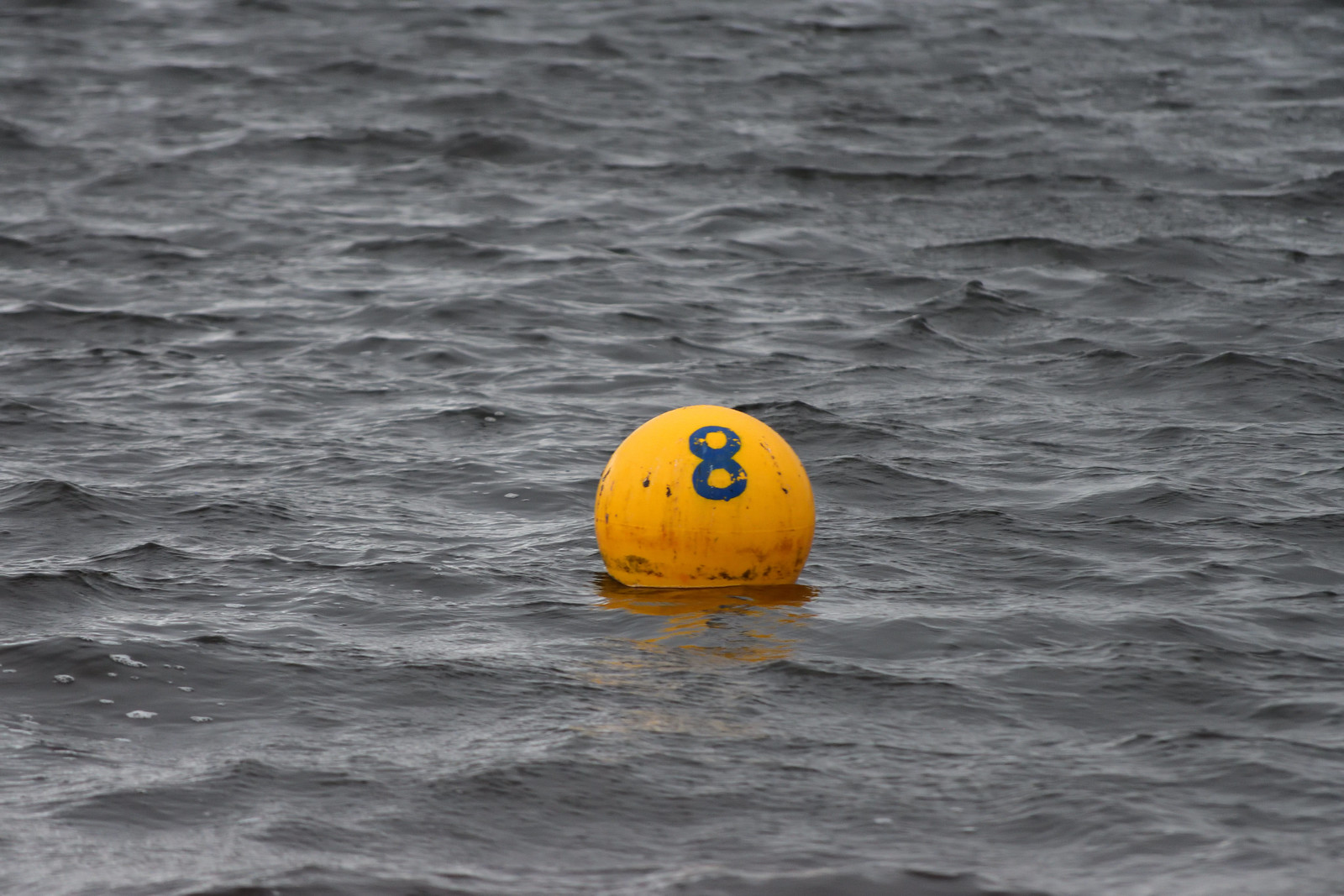The photograph captures a solitary scene of a yellow ball floating on a ripply, grayish-dark body of water. The ball, roughly the size of a volleyball, stands out with a blue number 8 painted from the top to its middle. The surface of the water is slightly rippled, indicating gentle movement, with subtle reflections playing off its surface. The ball itself appears aged and dirty, with distinct black stains around its bottom and scattered blue dots that almost resemble a face upon closer inspection. The entire composition centers on this floating ball amidst the vast expanse of water, evoking a sense of isolation and calm.